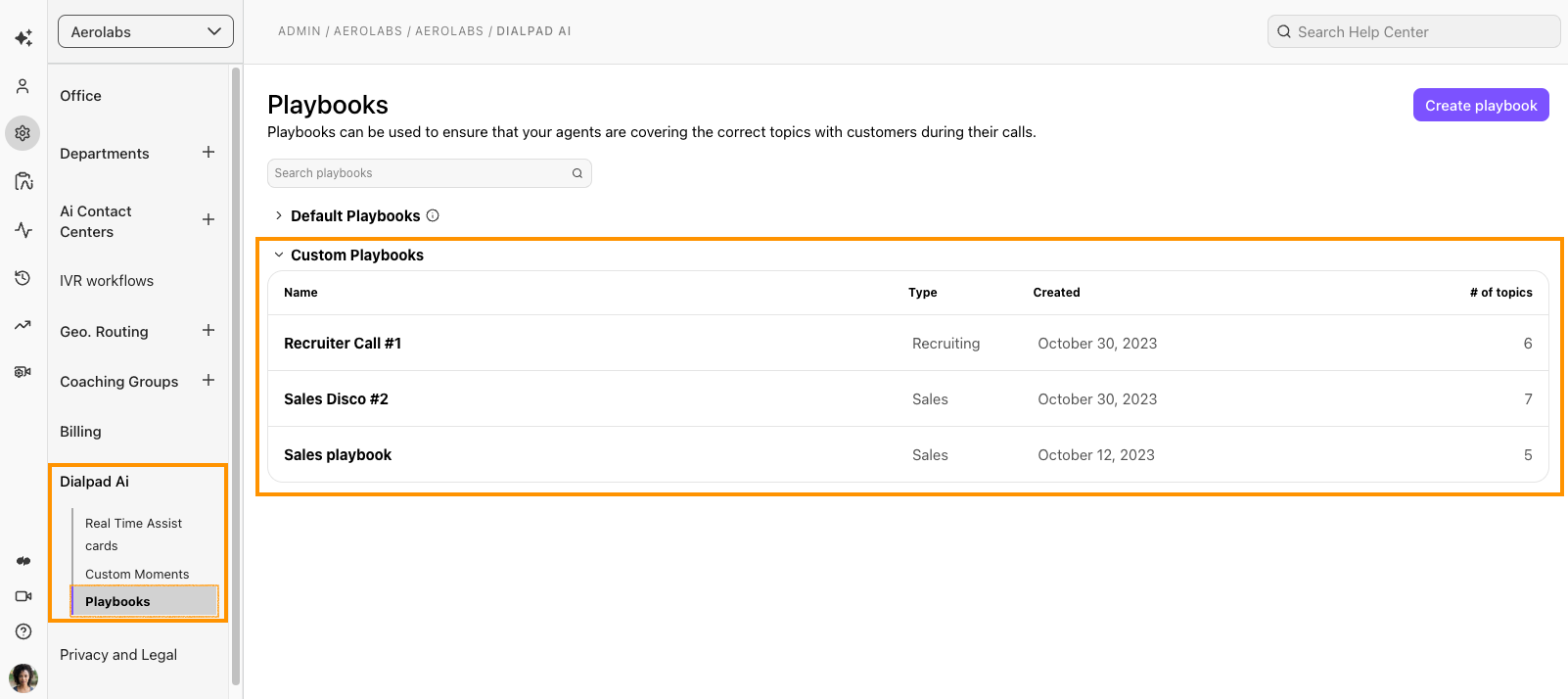This detailed and sophisticated caption provides a comprehensive overview of a user interface, highlighting key elements and their layout:

---

In the top-left corner of the interface, there is a drop-down menu labeled "AeroLabs." To its right, several tabs are separated by forward slashes: "Admin," "AeroLabs," and "Dialpad AI." On the top-right corner, there is a "Search Help Center" input field accompanied by a magnifying glass icon. Just below this, the section is titled "Playbooks." Here, it elaborates how Playbooks can be utilized to ensure agents address the correct topics with customers during their calls. Adjacent to this description, there's a button within a rounded rectangle labeled "Create Playbook."

Beneath the main Playbooks section, on the left-hand side, lies a "Search Playbooks" input field, which is currently grayed out. Below this input field, there is a section titled "Default Playbooks," featuring a right-facing arrow next to the title. Underneath, an orange-lined, rectangular dropdown labeled "Custom Playbooks" is displayed. 

Following the "Custom Playbooks" section, there is a list of playbook names: "Recruiter Call Number," "Sales Disco Number," and "Sales Playbook." Adjacent to each name are columns categorized as "Type," "Created When," and "Number of Topics."

Returning to the top-left corner below the AeroLabs dropdown menu, the interface lists multiple sections: "Office," "Departments" with a plus sign, "AI Contact Centers" with a plus sign, "IVR Workflows," "GeoRouting" with a plus sign, "Coaching Groups" with a plus sign, and "Billing." A square with orange lining denotes "Dialpad AI," followed by "Real-Time Assist Cards," "Custom Moments," and the highlighted and bolded option, "Playbooks." Finally, at the bottom of this list, there are options labeled "Premise C" and "Legal."

---

This caption ensures a precise visualization of the interface layout and features for the reader.